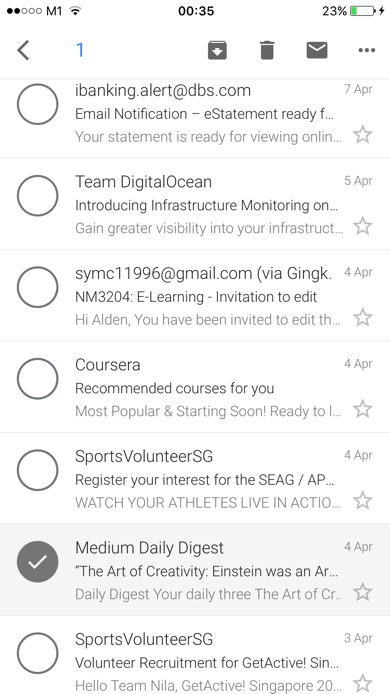Screenshot showing an email application on a smartphone screen. In the upper left corner, the connectivity status is displayed with a Wi-Fi icon. The upper right corner shows the battery level at 23%. The time at the top reads 12:35 a.m. Below, seven emails are listed, each accompanied by a circle. The sixth email has its circle filled in with a white check mark in the center, highlighting it in light gray. The email's subject reads, "Medium Daily Digest: The Art of Creativity Einstein Was", dated April 4th. A small star icon is positioned below the date. Above the email list, from left to right, there are icons for saving, trashing, and mailing, followed by a menu icon represented by three vertical dots.